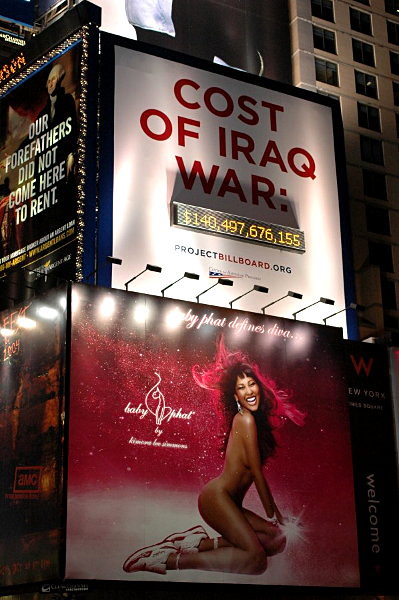The image captures four prominent billboards mounted on the side of a building. The top left billboard features a compelling historical message: "Our forefathers did not come here to rent," accompanied by a classic portrait of George Washington. To its right, another billboard powerfully protests the financial cost of the Iraq War, displaying the staggering figure: "$140,497,676,155" and directing viewers to "projectbillboard.org" for more information. Below these, the third billboard showcases a fashion-oriented advertisement with the slogan, "Baby Phat Defines Diva," promoting the "Baby Phat" brand. Each billboard captures a distinct message, blending American history, socio-political commentary, and contemporary fashion.